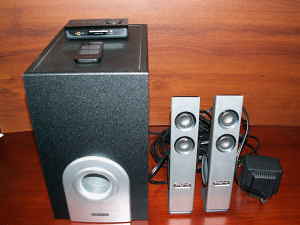This photograph showcases an indoor audio system featuring a large, black, rectangular subwoofer and two smaller, silver, rectangular speakers, all positioned on a wooden surface with a matching wood grain backboard. The subwoofer, prominently placed on the left, has a semicircular silver design on the bottom front panel and a small, unidentified device resting on it, possibly a card reader or a remote. Beside it, the two silver speakers have dual circular dark gray components for sound output and are connected by visible black wires. Behind these speakers, a noticeable box-shaped power adapter is plugged in. The wooden surface and the wall have distinct wood textures, with the floor being a darker shade of wood and the backboard a lighter, yet still dark brown, wood grain.